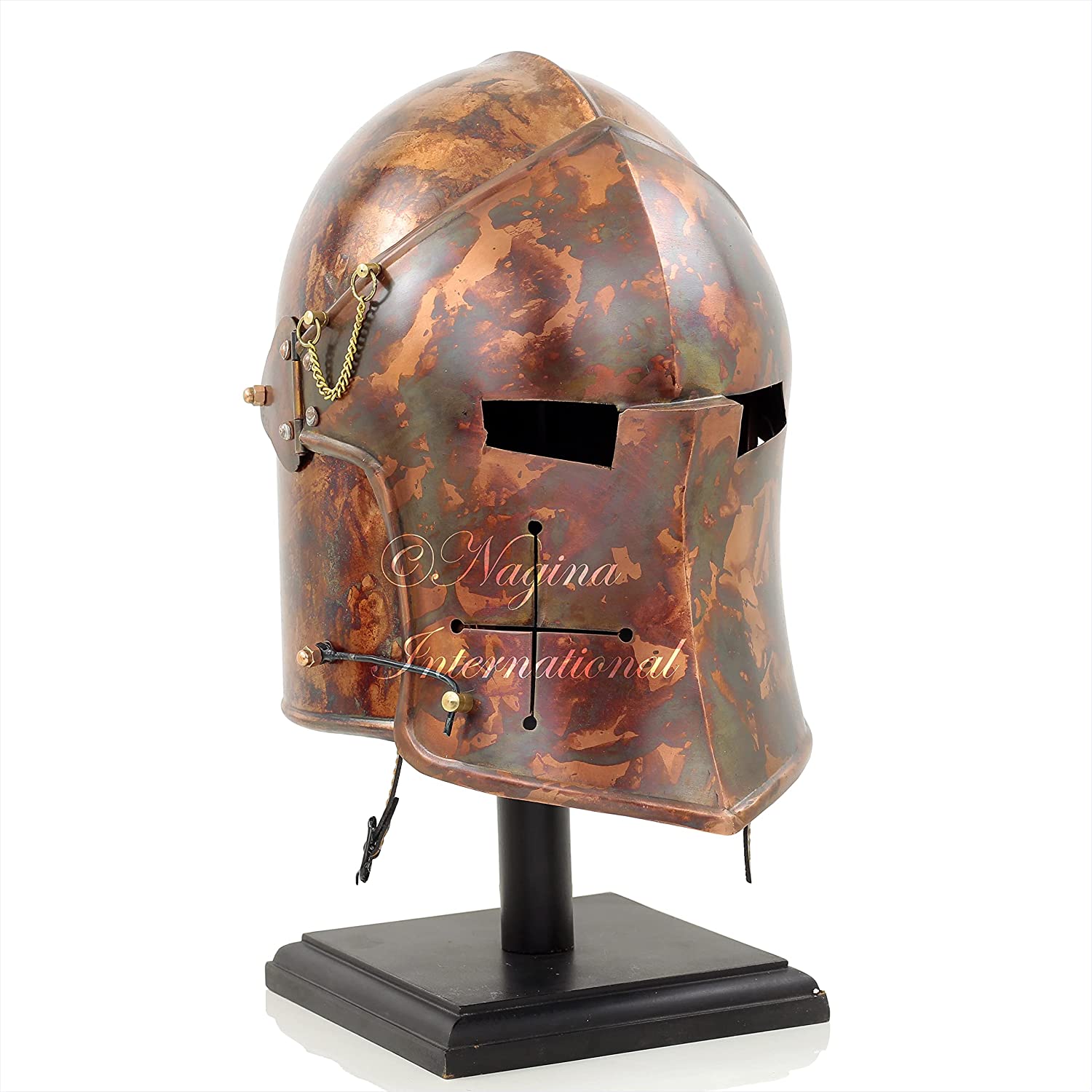The image depicts a battle helmet, bronze in color with hints of dark copper and lighter orange splotches, suggesting some age or rust. The helmet, which appears to be a full face covering extending possibly to the neck, features rectangular eye slits and a rounded top. It is displayed on a black wooden base and attached firmly via a central black support. A distinctive gold chain runs from ear to ear, possibly intended for decorative or functional purposes. Additionally, a watermark inscribed with 'Nagina International' is visible on the image. The backdrop is a plain white, enhancing the focus on the helmet's intricate details and slightly weathered appearance.